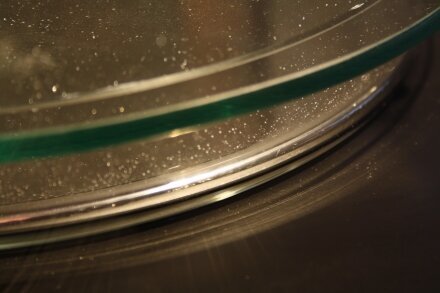The image features a close-up shot of a dark wooden table, potentially chestnut or very dark brown in color. Atop the table, there are several round objects that appear to be dinner serving chargers or plates. These chargers are predominantly dark brown, though they have unpolished, dusty silver or gold-colored rims. In the lower right-hand corner of the image, the table and objects cast a deep, dark brown shadow. The left and top sides of the photograph give the impression of looking through a dirty piece of glass. Near the center of the image, there is a noticeable glint, akin to sunlight reflecting off a gold-trimmed edge, casting rays that appear to illuminate the surfaces. While the bottom plate reflects light, adding a slightly shiny contrast, the top plate appears darker and possibly shows the shadow of the person who took the photograph.